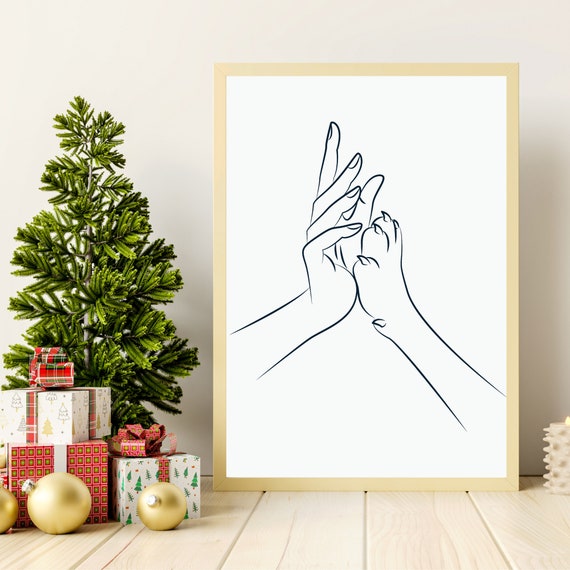In this photograph of a drawing, the scene is set against a light tan wall, with a light-colored, slatted hardwood floor. The main focus is a large, framed line drawing, possibly around two to three feet tall. This drawing, featuring a simple black sketch of a human hand high-fiving a dog's paw, leans horizontally against the wall. To the left of the drawing, there is a small, undecorated evergreen tree, resembling a modest Christmas tree. In front of this tree are three wrapped Christmas gifts: one adorned with Christmas tree wrapping paper and a red bow, another in red wrapping paper with a white bow, and the topmost gift wrapped in white paper with gold Christmas trees and a red bow. In front of these gifts, three oversized, gold-colored Christmas tree ornaments are scattered on the floor. The overall scene gives off a festive yet minimalist holiday vibe.